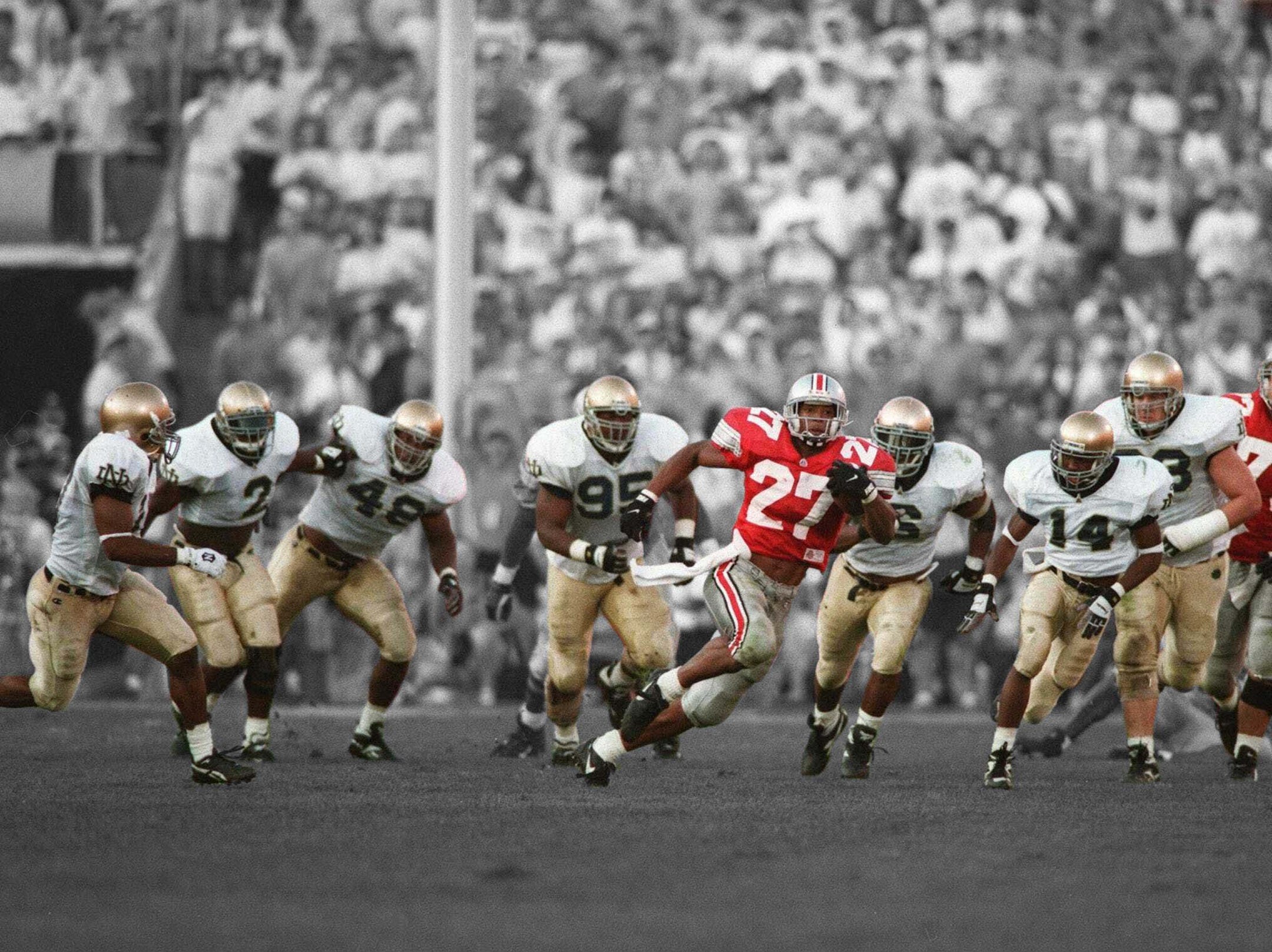This photo captures an intense moment from a college football game between the Notre Dame Fighting Irish and the Ohio State Buckeyes. In a striking visual contrast, the Ohio State running back, likely Beanie Wells, is seen charging down the field with fierce determination, gaining yardage while being chased by the entire Notre Dame defense. The Buckeyes' players are donned in red jerseys with white numbers and gray helmets adorned with red, white, and blue stripes, whereas the Fighting Irish wear white jerseys with black numbers outlined in gold, complemented by gold helmets and pants. Interestingly, this action-packed scene is the only element in color; the background, including the field and the cheering crowd in the stadium, is rendered in black and white, giving the photo a nostalgic, timeless feel. Among the players, various numbers such as 2, 14, 27, 48, 95, and partial numbers 3 and 6 are visible, adding to the detailed chaos of the chase.